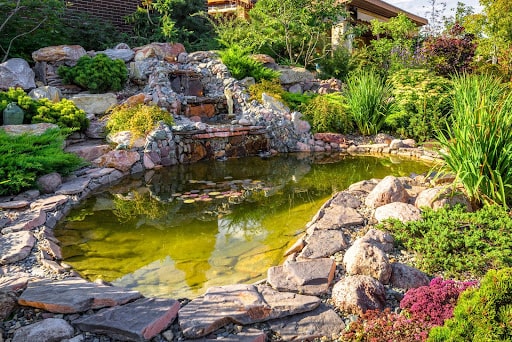This outdoor photograph captures a meticulously crafted backyard water garden featuring a small, man-made pond adorned with moss and multicolored lily pads, giving the water a greenish tint. The pond is circled by flat rocks and gravel, with an array of colorful vegetation including pink flowers, cattails, ferns, and various shades of green foliage like evergreen shrubs and yellow plants. The centerpiece of this scene is a decorative, multi-level waterfall. The waterfall, built with smaller rocks and extremely heavy boulders that would require machinery to move, cascades down to a rock-lined pond. Intricately placed amongst these boulders are steps, small statues on the second and third levels of the waterfall, and rich, red and green plants. The backdrop is lush with shrubs, flowering plants, and tall trees which nearly obscure a white house with a brown eave and a brick wall, hinting at the periphery. Boulders, rock gardens, and well-integrated planting create a harmonious natural setting enhanced by a patch of blue sky, adding to the peaceful ambiance of this beautifully maintained garden.